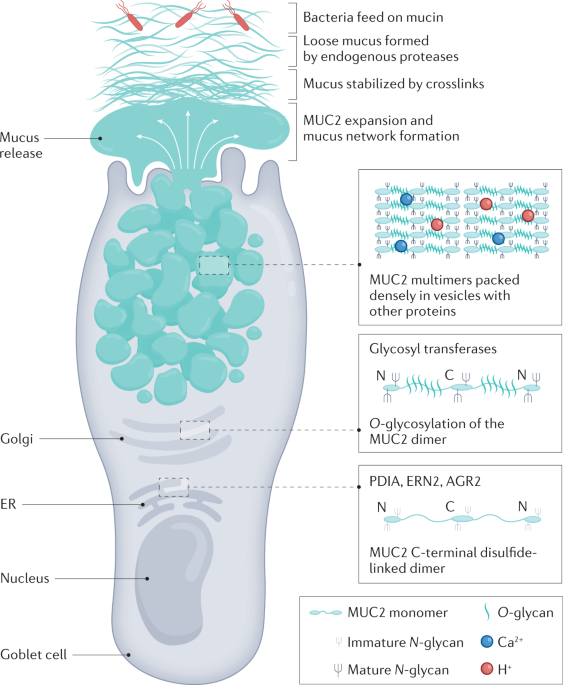This detailed scientific diagram illustrates the mucosal processes involving a goblet cell, prominently displayed on the left side of the image. The large, light gray goblet cell structure showcases various components such as mucin release, golgi bodies, and the endoplasmic reticulum (ER), with the nucleus centrally located. The goblet cell is engaged in mucin production, visible through numerous arrows pointing to specific cellular processes, including glycosyltransferases and other biosynthetic pathways. 

The diagram highlights key processes: "Bacteria feed on mucin," "Loose mucus formed by endogenous protease," "Mucus stabilized by cross-links," "MUC2 expansion," and "Mucus network formation." Mucin secretion is vividly depicted with blue, irregularly shaped circles emanating from the goblet cell, indicating the mucus release and formation. Insets on the right provide magnified views and black text boxes detailing specific cellular activities and structures related to mucus formation and stabilization. This comprehensive depiction serves as an educational resource, detailing the complex interactions and processes within a goblet cell related to mucosal biology.